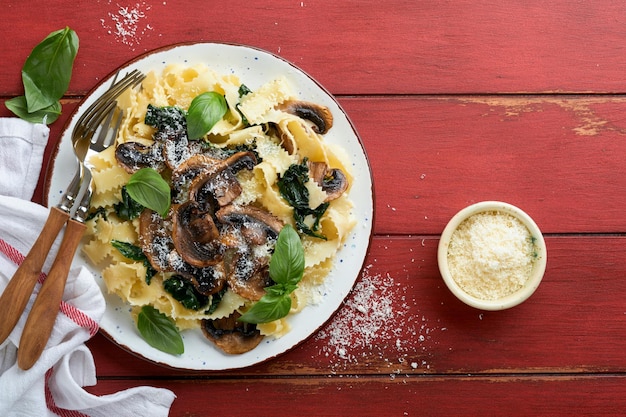On a weathered red wooden picnic table, there sits a simple yet appetizing pasta dish. The dish features wide, flat noodles with zigzag edges, similar to linguine but slightly wider. These noodles are topped with sautéed brown mushrooms and adorned with fresh whole basil leaves. A generous sprinkling of freshly grated Parmesan cheese completes the dish, with some of the cheese also scattered around the white plate and on the table. The plate, accented with gold trim, is paired with two forks—one placed atop the other, their handles crafted from wood. Beside the plate is a white napkin featuring a red stripe pattern. To the right of the plate, in a small white bowl, lies extra Parmesan cheese. The rustic setting and thoughtfully arranged elements suggest this is a professionally styled food photo, perhaps intended for a food blog or culinary magazine.